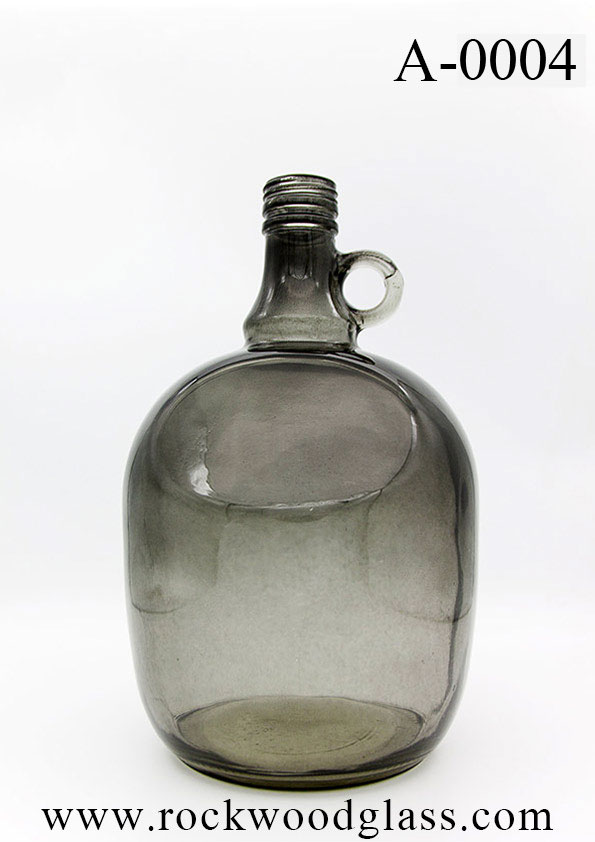This image is an advertisement for Rockwood Glass, featuring a prominent glass jug as its central element against a solid white background. In the top right corner, black text reads "A-0004." The jug itself is large and bulbous, predominantly dark grayish with a transparent quality, allowing visibility through it despite its stained appearance. It features a small top with a very small handle, a circular opening in the front evoking the style of old-fashioned glass Coca-Cola bottles, and a loop on the side, possibly serving as a finger holder. On the bottom of the image, the company's website, "www.rockwoodglass.com," is displayed in black lettering.